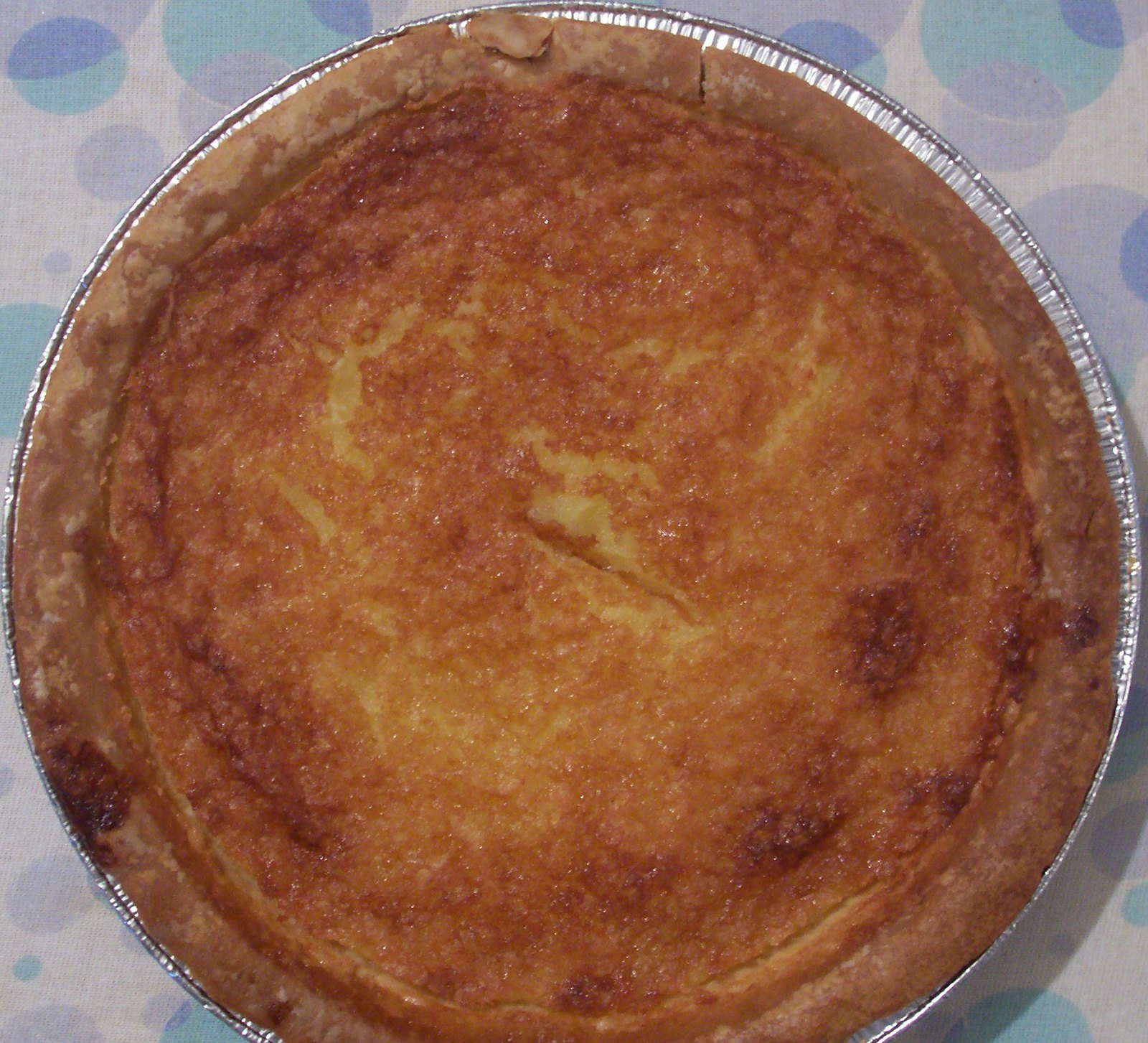This color photograph, square in format, captures a delectable pie placed on a light cream background adorned with pale blue and purple circles. The pie, primarily centralized but slightly cropped at the bottom, rests in an aluminum foil pan with its silver rim visible. The pie features a dark brown, golden crust and a bubbly, browned custard top, suggesting a well-baked texture. A knife slit is visible at the center of the pie, indicating a check for doneness. Some of the custard has slightly pulled away from the crust's edge, enhancing its homemade appeal. This realistic food photograph embodies a detailed and appetizing representation of a sweet, creamy pie.